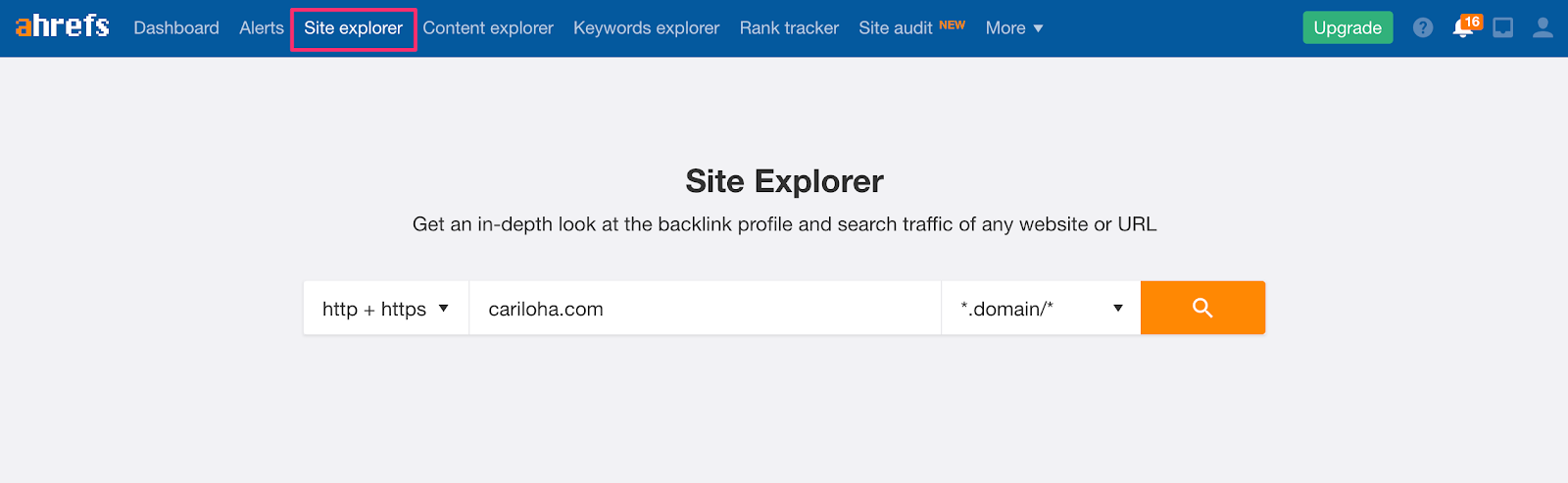The image features a blue background with a significant amount of detail geared towards SEO analytics. At the top, a dark blue box contains the logo "Ahrefs", with the letter 'A' highlighted in red while the rest of the letters are in white. Below this, there is a navigation bar including sections such as "Dashboard," "Alerts," and "Site Explorer," the latter highlighted with a red box. Additional sections listed are "Content Explorer," "Keywords Explorer," "Rank Tracker," and "Site Audit," with the word "New" in red beside it, followed by "More" accompanied by a down arrow. 

To the right of these options, a prominent green button labeled "Upgrade" stands out, followed by an icon of a bell with a red square indicating the number 16. 

In the central part of the image, over a light blue background, the "Site Explorer" feature is highlighted with the text: "Get an in-depth look at the backlink profile and search traffic of any website or URL." In this section, there is a dropdown option between "HTTP" and "HTTPS," followed by an input field containing "caraloa.com" with another dropdown option to choose the domain. A magnifying glass icon in an orange box signifies the search function for this tool.